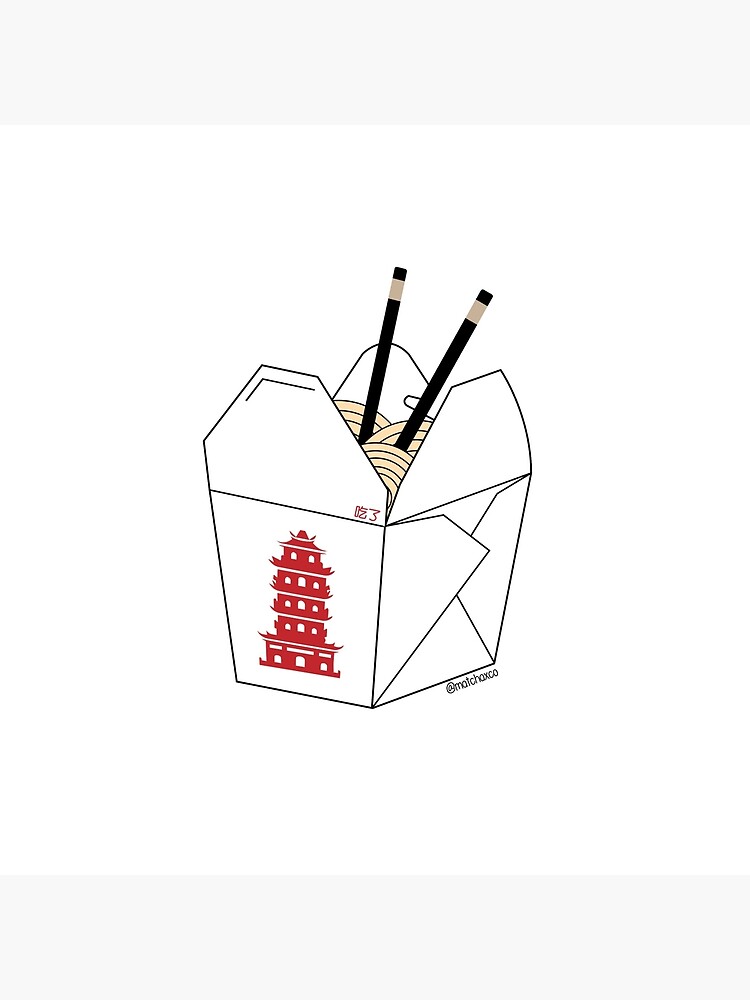The image is a detailed, cartoon-like color illustration of a traditional Chinese takeout box, portrayed in a square format with a white background. The white, trapezium-shaped box has black outlines and three tabs that are open, revealing a pile of yellow noodles inside. A pair of black chopsticks, featuring a cream-colored band near the top, protrude from the noodles, angled toward the upper right corner of the image. The front of the box, which is facing the bottom left of the illustration, displays a red, five-story pagoda-style tower with three white windows per floor, except the top floor which has two windows. The tower's base on each floor is tilted slightly upwards. Additional visual elements include light gray horizontal bars above and below the box. The word "Machaxko" is written below the illustration, which is bordered by overlapping cardboard on the sides.